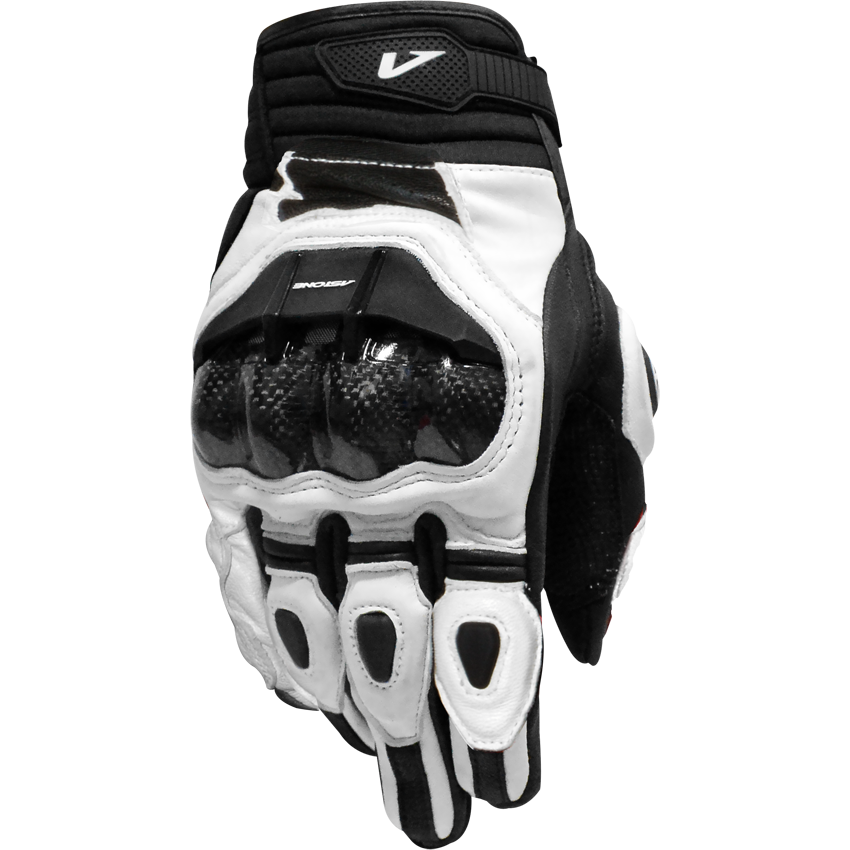This image showcases a high-quality, black and white glove designed for extreme sports, possibly motocross or snowboarding. The glove features a combination of materials, including white leather and black mesh, enhancing both durability and flexibility. The fingertips are well-padded while allowing movement, and the knuckles are reinforced with hard black plastic shields for extra protection. The glove also sports a black thumb with an added protective patch and a shiny black section over the back of the palm. The wrist strap, which bears the letter "V," is elastic and adjustable, ensuring a secure fit. Set against a clean white background, this close-up product image emphasizes the glove's construction and protective features, suggesting it's intended for vigorous sporting activities.